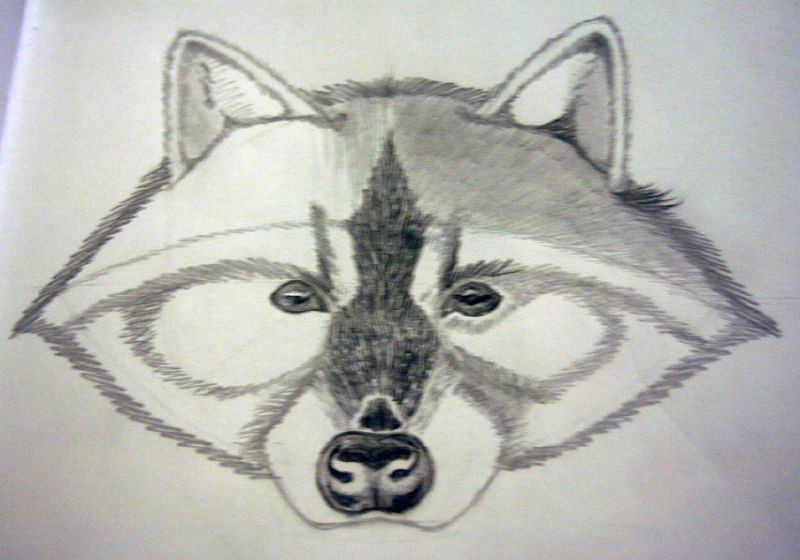This image captures a detailed photograph of a raccoon drawing, evidently created as a practice exercise in sketching and shading techniques. The raccoon’s head is notably broad, resembling the shape of a football, which serves as an apt description of its overall form. Distinctive triangular ears with well-defined inner ear details exhibit careful attention to anatomical accuracy. There is a noticeable gap followed by nuanced shadowing within the ears, indicative of a focus on realism.

Shadowing practice is evident throughout the drawing, adding depth and dimension to various parts of the raccoon's face. The creature’s pronounced black nose stands out, although the mouth remains unseen. The eyes are encircled by multiple lines that give character to the raccoon, complemented by a substantial black stripe running from the nose to the top of the head.

The raccoon's facial coloration is intricately managed; the entire top right side of its head is shaded a darker gray, contrasting sharply with the pristine white of the left side and most of the lower face. This asymmetry in shading suggests that the artist might be experimenting with lighting effects or perhaps is in the midst of completing the shading process. Overall, the image captures a work-in-progress drawing that showcases foundational skills in raccoon illustration and shading techniques.